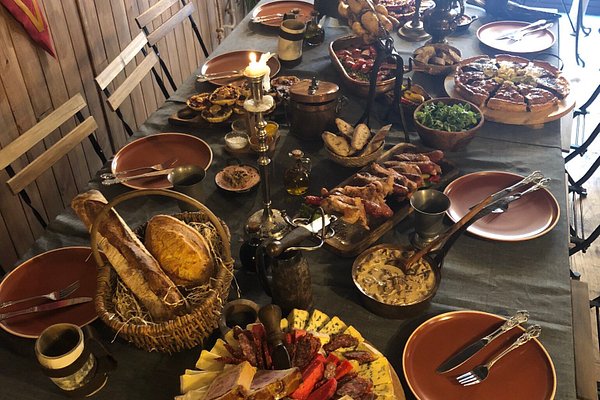This color photograph captures a cluttered dining table set meticulously for a meal. Dominating the scene are numerous food items, including a charcuterie board partially out of frame, a skillet containing dip, a platter of chicken, and two bread baskets—one with whole loaves and another with smaller pieces of bread. The table also features two salads, a possible tart or Chicago deep-dish pie, and a variety of cheeses and meats. Brown round plates complete with forks and knives are arranged angularly, ready for use. Drinkware on the table includes a beer stein and a copper glass, accompanied by a carafe of oil. Centered on the table is a tall candlestick with a nearly burned-down candle, casting a soft glow over the spread. The background reveals three wooden chairs and a wooden wall, adding a rustic touch to the setting. An ambiguous red, pointed object hangs from the top left corner, adding an element of curiosity to the image. The absence of people focuses the attention on the abundant and diverse assortment of food, suggesting a hearty meal about to commence.